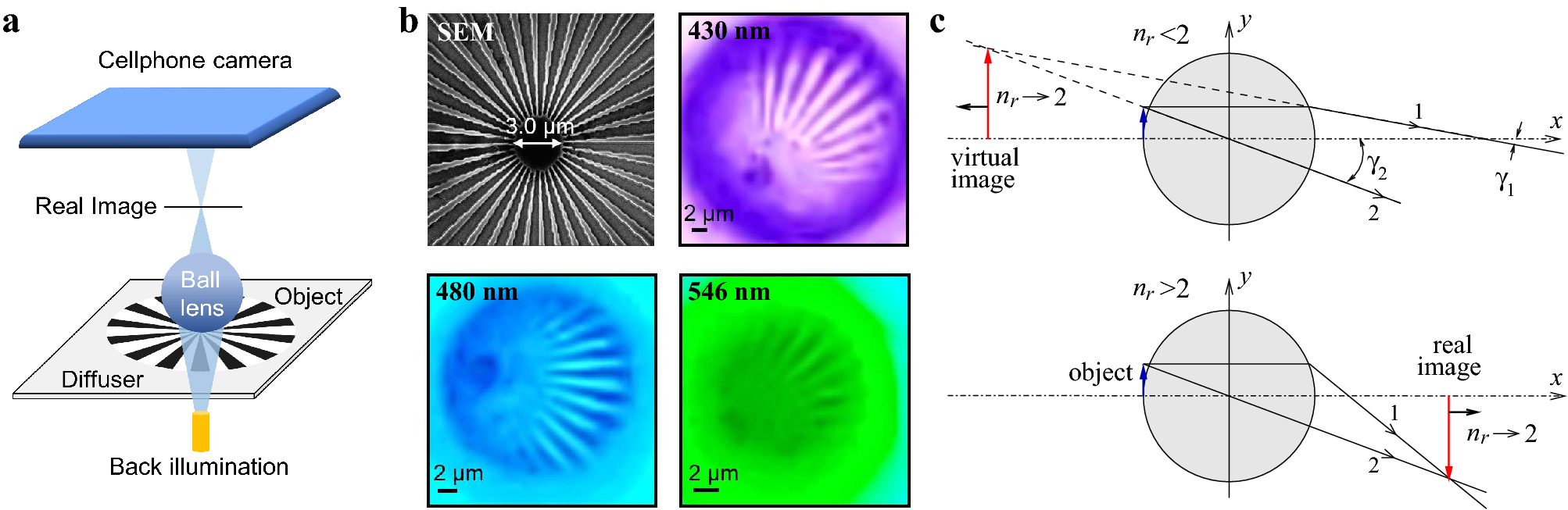The image presents a complex array of shapes, equations, and illuminated text, primarily appearing against a white background. Centered within the image are two distinct configurations: a grid of two-by-two circles and lines in various neon colors, including purple, blue, green, and other hues such as gray, white, red, black, and orange; and on the far left, there are two squares with a ball positioned between them. The right third of the image features more circles and lines, overlaid with mathematical equations such as "n sub r to 2." Prominent text within the image includes terms like "cell phone camera," "back illumination," "real image," "virtual image," and references to specific wavelengths (430 nm, 480 nm, 546 nm). Additional annotations such as "SEM," "BSEM," and other descriptive words help depict a detailed scientific or mathematical visualization using various shapes and colors to distinguish different elements and concepts.